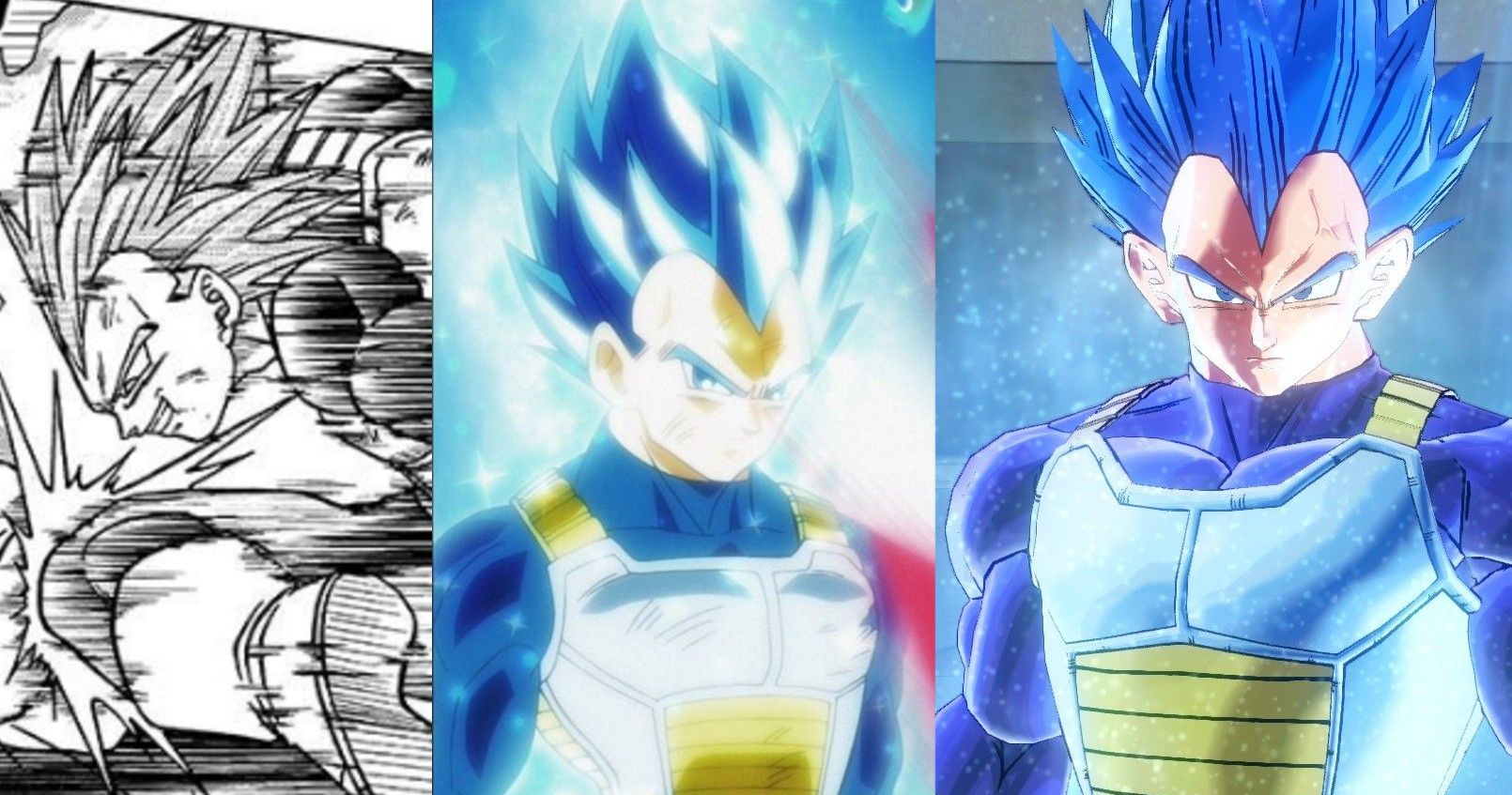This triptych features three evolving portraits of a character, likely from a comic book or video game, with strong indications pointing toward the Dragon Ball Z franchise. On the far left, the image is a black-and-white sketch, showing the character in a slightly hunched posture with a menacing expression and wild, long spiky hair. The middle panel presents the same character in vibrant colors, with tall, spiky blue hair and a scowling face. He wears a dark blue shirt beneath a light blue and gold body armor, set against a light blue and white background. The rightmost image reveals the character again, now with a clearer and more pronounced depiction. His spiky blue hair towers over his angry face, and his muscular build is emphasized by the dark blue uniform and the light blue and gold shield-like armor over his chest. The background remains consistently light blue, enhancing the cohesive yet dynamic representation of this fierce, iconic fighter.